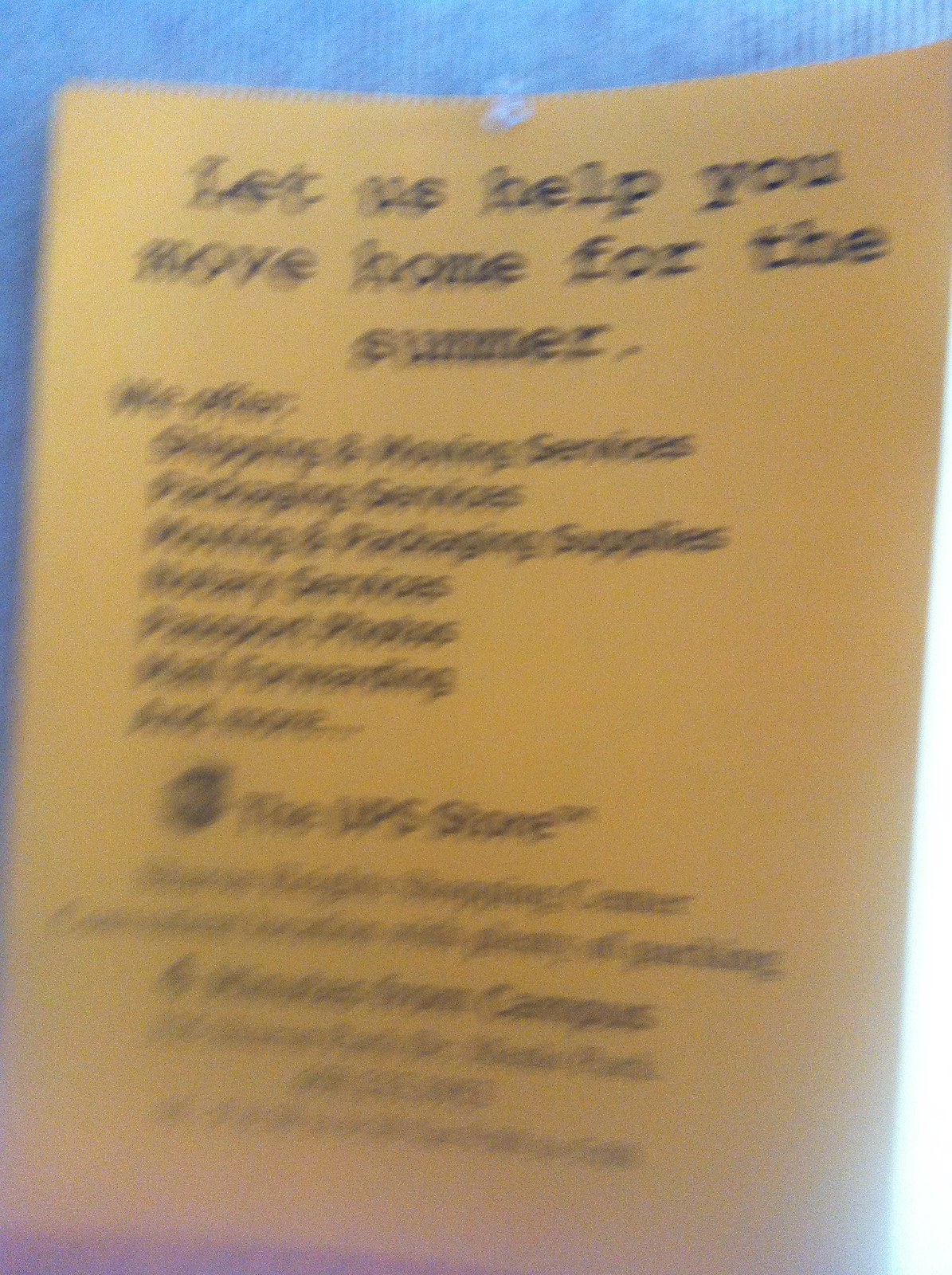Captured in a hurried moment, this blurry, low-resolution image showcases a flyer for a moving service. The flyer, printed on goldish yellow paper with black font, bears the slightly blurred message: "Let us help you move for the summer." The listings on the flyer include a range of services such as shipping, moving, packing, packing supplies, notary services, passport photos, and mail forwarding. The flyer promotes the UPS Store and provides an address, though it remains indistinct due to the photograph's poor quality.